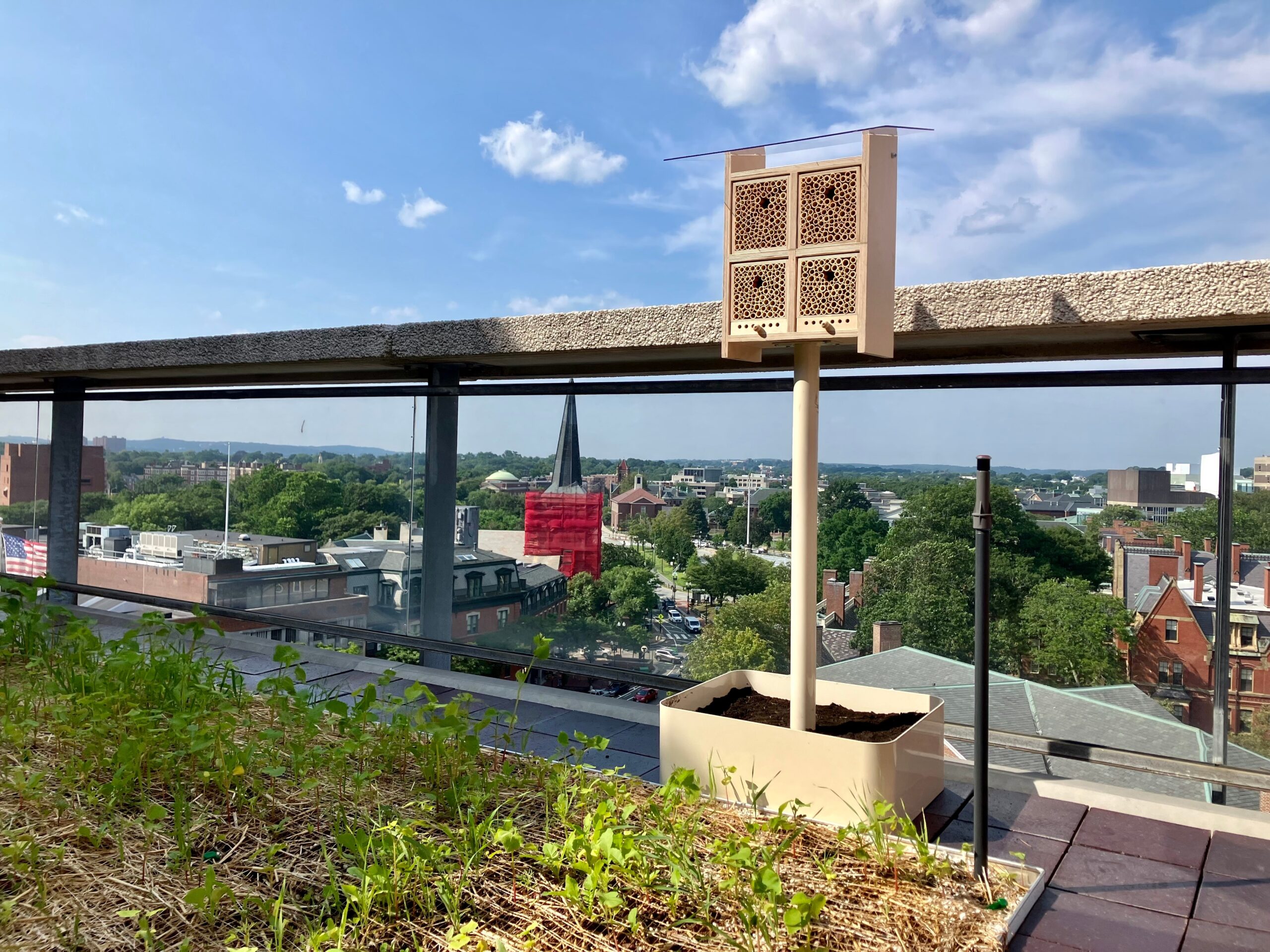The photograph, taken outdoors during the daytime, captures an elevated balcony scene with a detailed view of a town in the background. The balcony itself is bordered by a railing constructed from a combination of glass and steel bars, topped with cement. At the forefront of the image, there is a small makeshift vegetable garden featuring shoots of green leafy plants and weeds emerging from light-colored straw.

A bird feeder, possibly also used as a bat house due to its design, stands out in the center of the garden. It is mounted on a long pole and comprises a large square structure with four smaller squares, each containing honeycomb-like holes for birds or bats to access seeds. Nearby, the garden area is contrasted by dark gray rectangular stones forming a walkway.

In the background, the town is visible with various brick buildings and a distinctive structure with a green, rustic steeple and red scaffolding, likely a church. The townscape is highlighted by a mix of green trees and additional buildings. A notable feature in the background is a concrete structure elevated on gray cylindrical columns, its purpose unclear.

Above, the sky is a mix of blue and white, partly cloudy. The sun shines brightly, casting light across the scene and creating a clear, vibrant atmosphere.